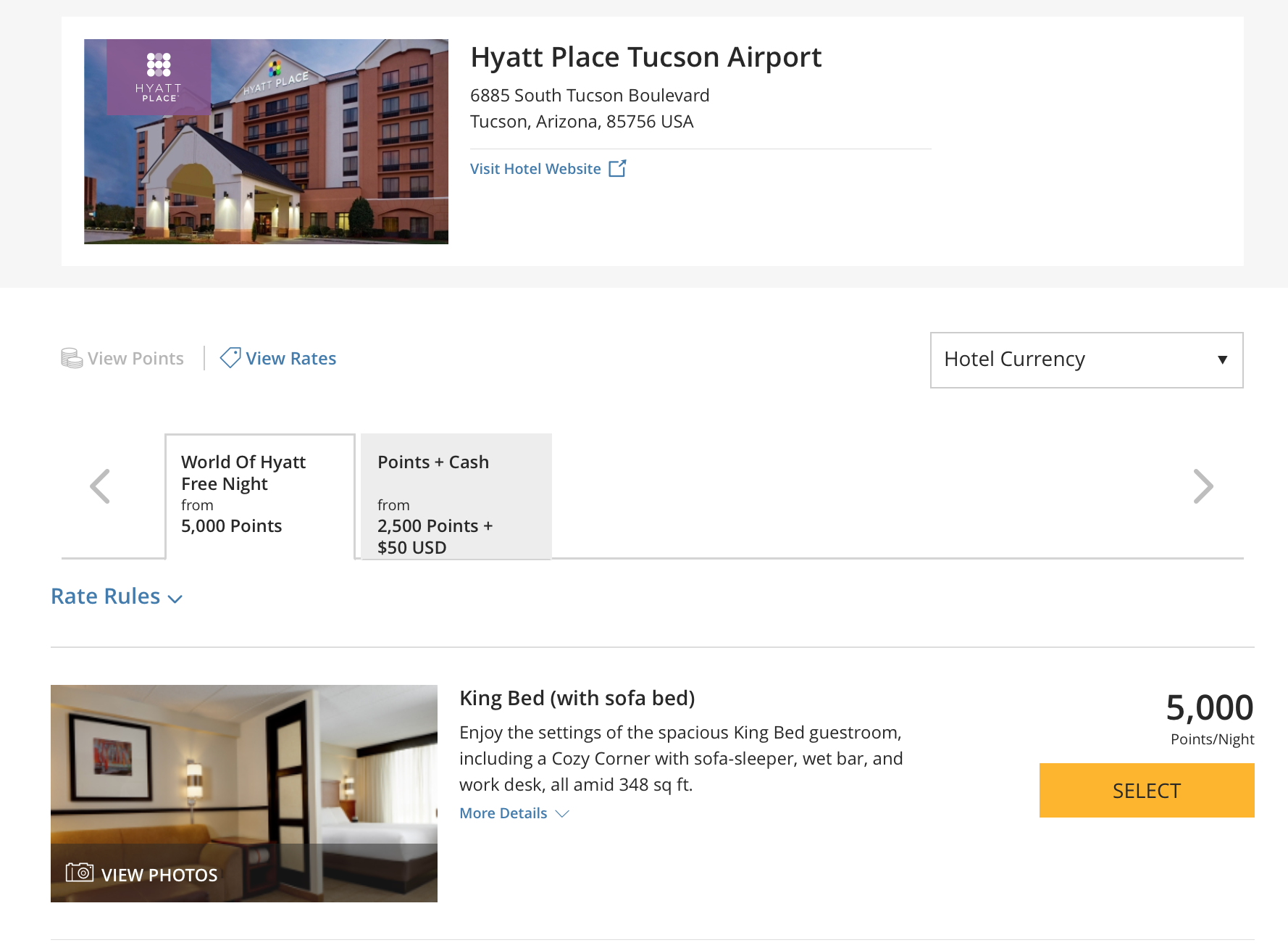### Caption:

The image showcases a comparative view of two different hotel options at Hyatt Place, Tucson Airport. At the top, a box prominently displays an exterior image of the Hyatt Place hotel located at 6885 South Tucson Boulevard, Tucson, Arizona, 85756, USA, with an accompanying link to visit the hotel's website. 

Below this, two primary options are presented: "View Points" and "View Rates," with the former grayed out and the latter highlighted in blue text. Adjacent to this, a drop-down menu labeled "Hotel Currency" is visible.

On the left side, two tabs are displayed, with the selected tab indicating "World of Hyatt Free Night from 5,000 points." Beside it, another tab reads "Points + Cash from 2,500 points + 50 USD". 

Beneath these tabs, an image illustrates the interior of a guest room. The room features a sofa on the left and, separated by a partial partition, a king bed on the right. The room description reads: "King Sofa (with sofa bed) - Enjoy the settings of the spacious king bed guest room, including a cozy corner with sofa sleeper, wet bar, and work desk, all within 348 square feet." On the right side, the rate is listed as "5,000 points per night," accompanied by a yellow "Select" button.